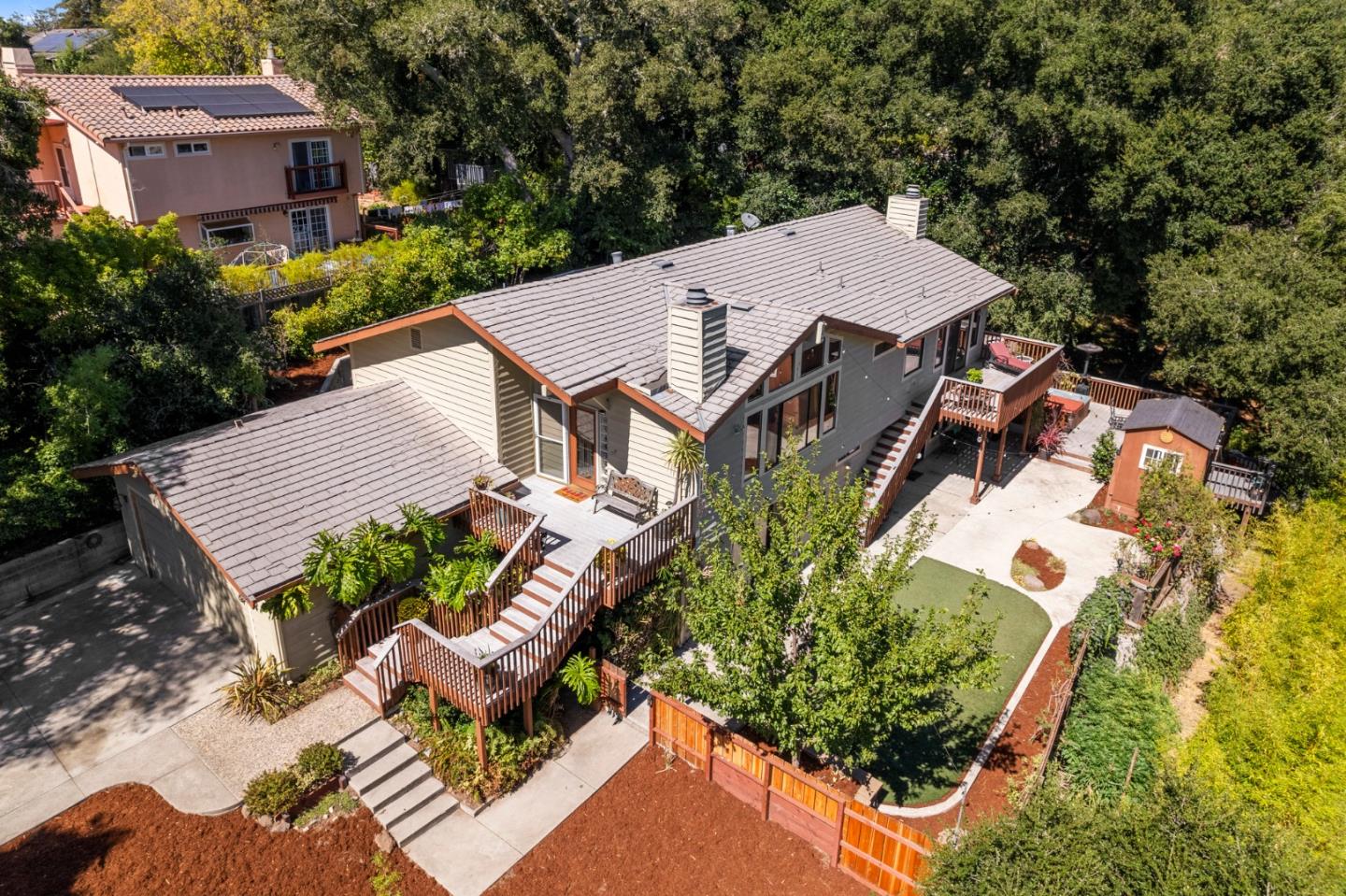This outdoor daytime photograph captures an elevated view of two houses set amidst a lush, well-manicured landscape. The prominent house in the center is a gray, two-story residence with a matching slanted gray roof that features two chimneys, one at the front and one at the back. The house has two distinct porches: the left-side porch with a chair and a right-side porch with a bench. Adjacent to the garage on the left, a driveway leads to a walkway that wraps around the garage and connects to stairs ascending to a balcony. This balcony has steps leading down to a footpath, which converges into a fenced concrete backyard area. This backyard features a wooden deck overlooking a wooded area, red mulch, and a combination of well-maintained gardens and towering trees.

Adjacent to this house, slightly higher up the hill on the left, is a second house with a unique pinkish hue and a slanted tiled roof adorned with black solar panels. The upper patio, framed by a black fence, overlooks the surroundings and hints at the modern amenities within. Both houses are complemented by verdant greenery, large trees of varying shades of green, and well-defined garden landscapes, giving the property a serene, inviting atmosphere. This photograph offers a comprehensive view ideal for showcasing the properties' features and the natural beauty of their settings.